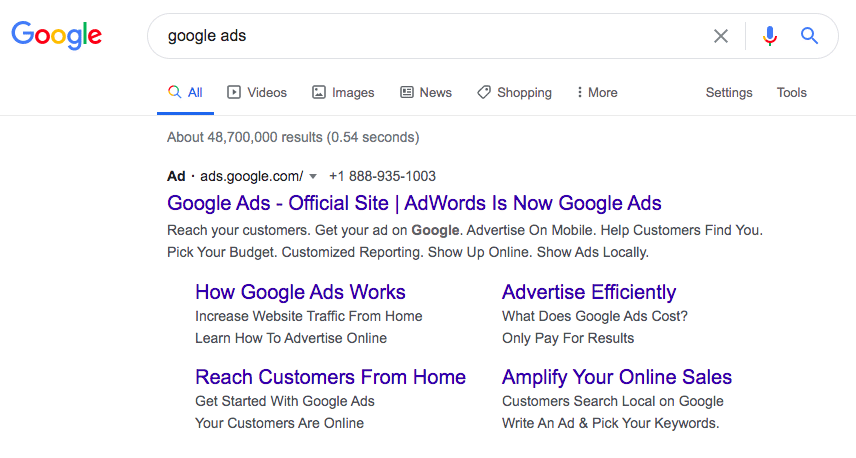This detailed caption describes a screenshot of a Google search result page for the query "Google Ads" displayed on a desktop screen. The topmost result is a sponsored advertisement by Google Ads, prominently showcasing the rebranding from "AdWords" to "Google Ads." The ad emphasizes various features and benefits of using Google Ads, such as reaching diverse customers, customizing reporting, and displaying ads locally. The advertisement includes a link to the official Google Ads site (ads.google.com) and provides a contact phone number (1-888-935-1003). Below the main ad, there are several links offering more information on topics such as how Google Ads works, how to reach customers from home, advertising efficiently, and amplifying online sales. These links appear to direct users to specific sections of the Google Ads website for further details.